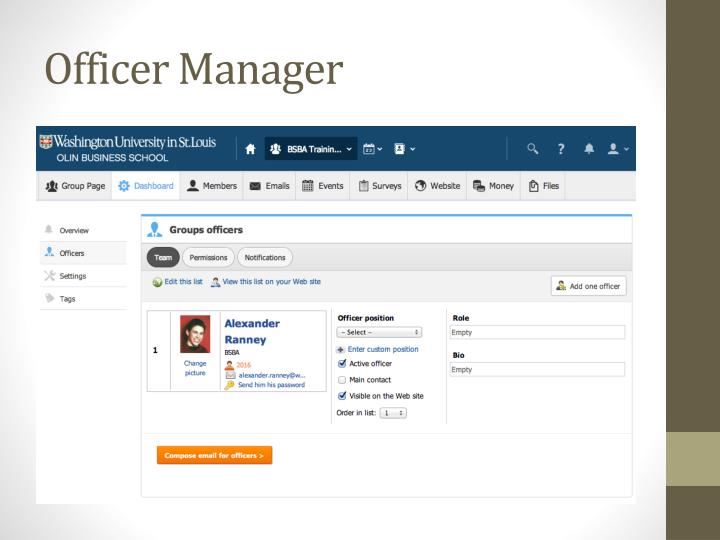The image depicts a presentation slide showcasing a screenshot of an online school website interface from Washington University in St. Louis Olin Business School. The screenshot is slightly off-centered and features a blue bar at the top highlighting the website's name. Below the bar, the interface is set to the dashboard tab, displaying information under "Group Officers" with a picture of Alexander Rainey and his details. The site has multiple navigation tabs including Group Page, Dashboard, Members, Emails, Events, Surveys, Website, Money, and Files. The slide itself has a vertical olive-brown bar running down its right side, and a slight gray gradient along the left side of the white background. The top text in large black letters reads "Office Manager," emphasizing the professional context of the content.